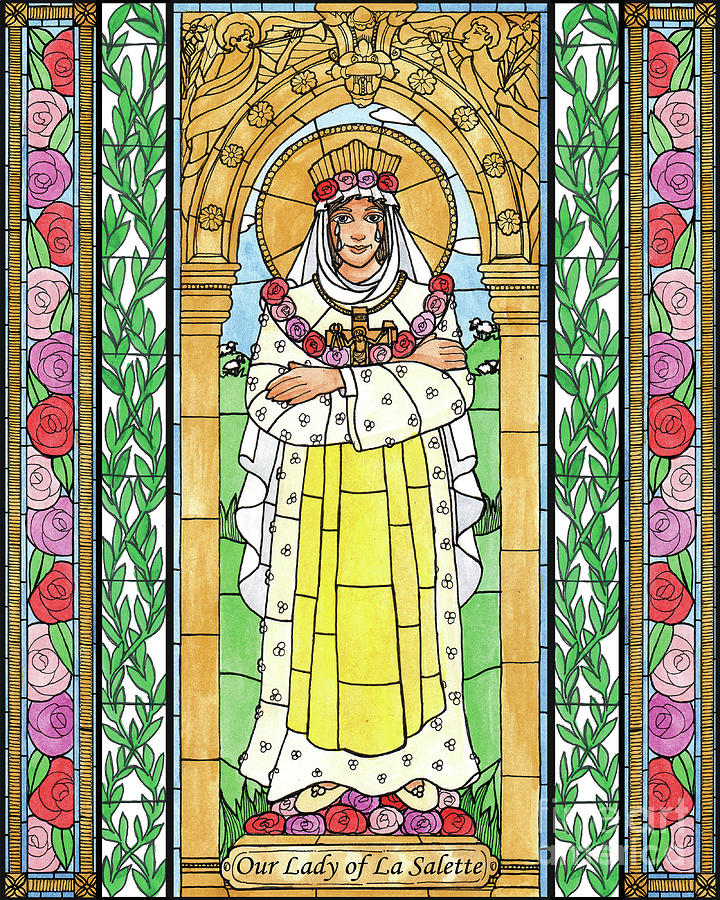This detailed caption describes a digital screenshot of an artwork resembling a painted stained glass depicting Our Lady of La Salette. At the bottom of the image, the script reads "Our Lady of La Salette," placed beneath her feet, surrounded by red, pink, and magenta roses. The lady stands solemnly at the podium, adorned in a flowing yellow robe with sections of floral patterns, complemented by floral sleeves and a white gown underneath. Her attire also features decorative elements such as a floral border, ruffles along the sides, white slippers, and a white veil with a headpiece of roses and a gold crown.

Our Lady's expression is serious, with visible teardrops streaming down her cheeks, adding an element of sorrow to her visage. Encasing her is a brilliant gold archway embellished with trumpeting angels and ornate floral decorations. Beyond this golden arch, green fields dotted with tiny sheep stretch into the distance.

Red and pink roses with verdant green leaves are prevalent throughout the image, with additional decorative elements flanking her neck and scattered at her feet. The entire composition, dominated by gold, red, pink, purple, and green hues, exudes a glowing pastel ambiance. The backdrop includes sections of white ferns and floral ornamentation, all contained within thin bamboo-like rectangular borders, enhancing the intricate and serene beauty of the piece.